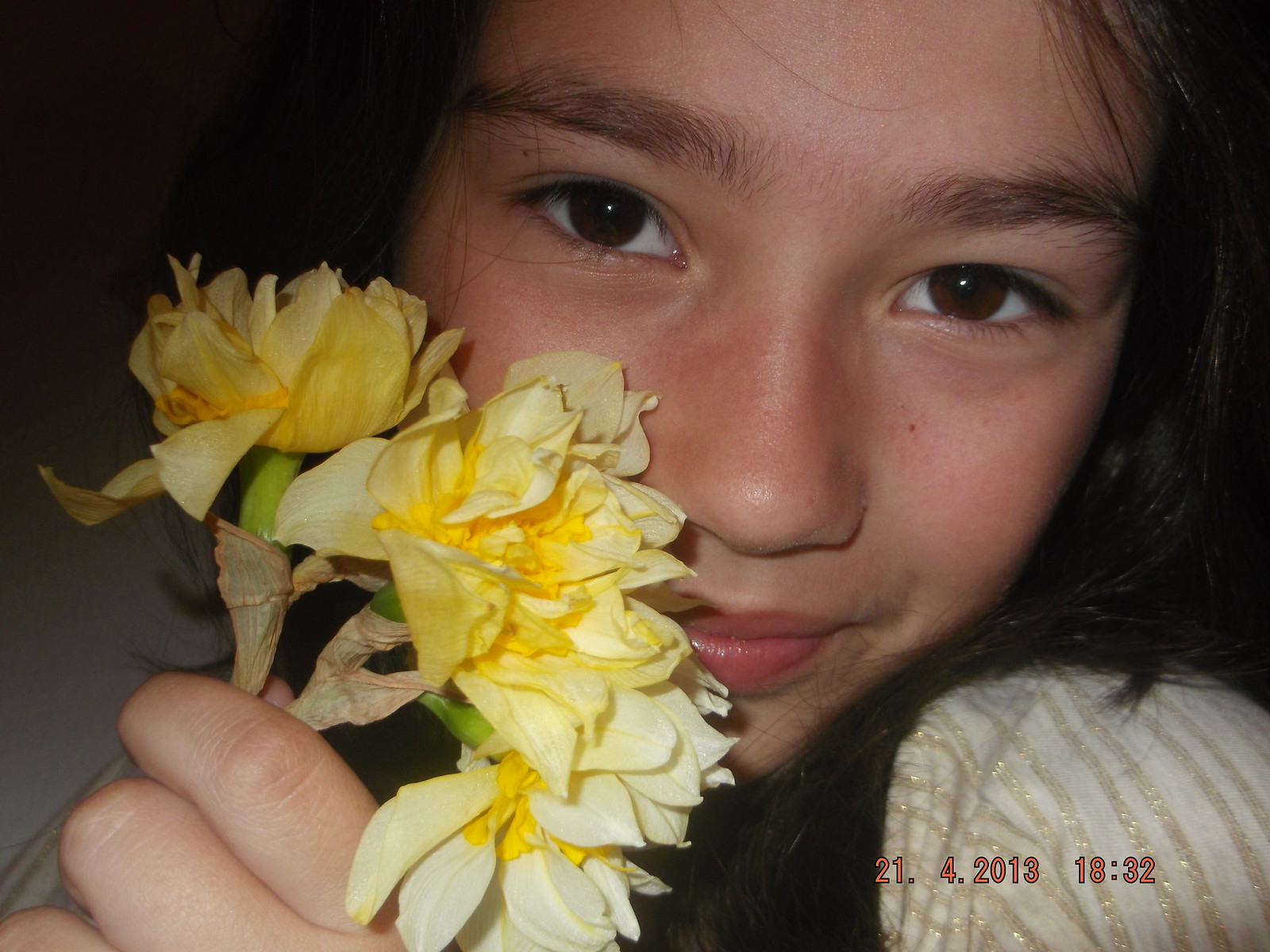A close-up image of a young girl with long, dark hair and dark brown eyes. She is wearing a white shirt adorned with golden stripes. She's smiling as she holds four yellow flowers with green stems, some of which have a tan husk. The flowers are positioned against the right side of her face. The time stamp "21.4.2013. 18:32" is visible in the bottom right corner of the image. The background is very dark, making it difficult to distinguish any details behind her. Her lips glisten with a hint of lip gloss, adding to her cheerful expression.